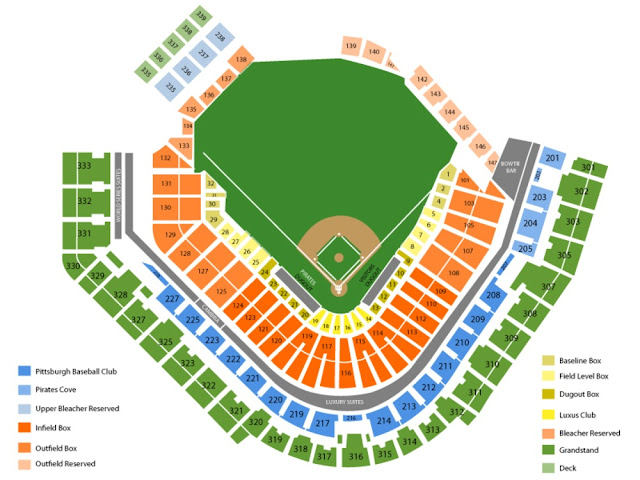A comprehensive and detailed image of a baseball stadium layout, showcasing various seating sections and amenities. The image prominently features the baseball diamond at the center, surrounded by an array of seats. Closest to the field are the baseline box and field-level box seats, offering optimal views of the action. As you move further back, the bleachers reserved and the grandstand seats are visible, marked in green. The Luxus Club seats stand out in orange, while the light green section delineates the deck.

The luxurious Pittsburgh Baseball Club, indicated in blue, is another notable seating area. The Pirates Cove, also in blue, provides an exclusive fan experience. Higher up, the upper deck seats offer a broad perspective of the game. Additional areas include the outfield reserved and outfield box seats, ensuring ample options for spectators.

Finally, several premium amenities are highlighted, such as the World Series Skates, the Bowtie Bar, and the Luxury Suites, catering to guests seeking a more upscale experience. Although the specific stadium is not mentioned, the detailed segmentation of seating sections presents a typical and standard modern baseball park layout.